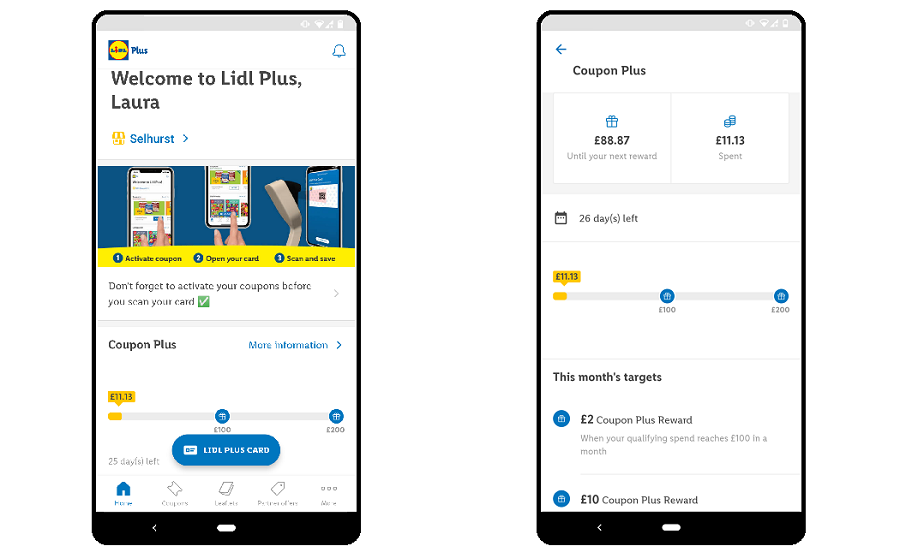**Descriptive Caption:**

This image features two detailed screenshots from the Lidl Plus app, highlighting user Laura's status and available actions. 

The first screenshot welcomes Laura with the message, "Welcome to Lidl Plus, Laura," and notes her location as "Sellhurst." Dominating the center of the screen is a large promotional image showing a hand pointing towards a coupon on a smartphone. Underneath this image, a series of instructional texts guide the user: "Activate your coupon, Open your card, Scan and save." Accompanying pictures illustrate the steps: opening the coupon, viewing the card selection, and scanning a QR code. Below this, a reminder in bold text urges, "Don't forget to activate your coupons before you scan your card." Additional information is indicated by a green checkmark and an arrow pointing right for more details. 

The bottom section displays Laura's progress with her Lidl Plus card: she has spent £11.13, progressing towards her halfway target of £100 and final target of £200. Her progress is indicated with a golden bar on the tracking meter, and she has 25 days remaining to reach her goal.

The second screenshot shifts focus to Coupon Plus, indicating Laura's exact figures: £88.87 needed until her next reward, with £11.13 already spent. It reinforces her time limit with "26 days left." This month's target offers a £2 reward upon reaching a £100 qualifying spend within the month. These targets and deadlines prioritize incentivizing Laura's continued engagement with Lidl Plus.